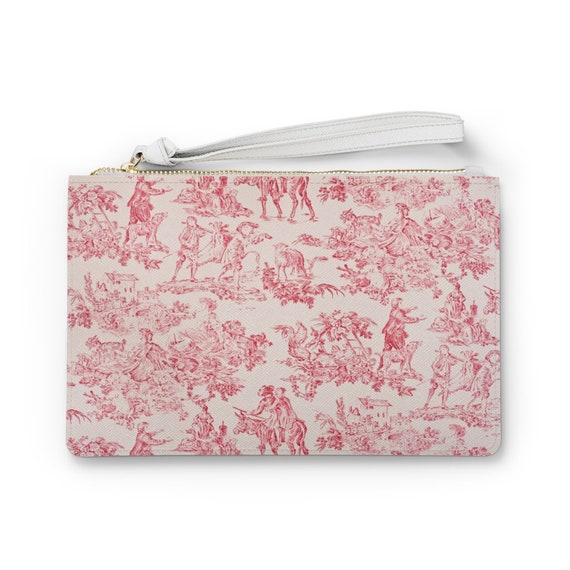This image features a small rectangular coin purse set against a white background, casting a shadow towards the bottom and right. The purse showcases a vintage-style design with intricate red illustrations on a cream-white fabric. The detailed prints include a monk on a donkey with two riders, a boy with his dog, a rooster, a sheep, various plants and leaves, a house in the distance, and floral patterns. The top of the purse features a white zipper with golden teeth, complemented by a gold ring. Attached to the zipper pull is a long white leather wrist strap, showing visible seams. The overall appearance combines a nostalgic charm with meticulous detailing, making it both functional and aesthetically pleasing.